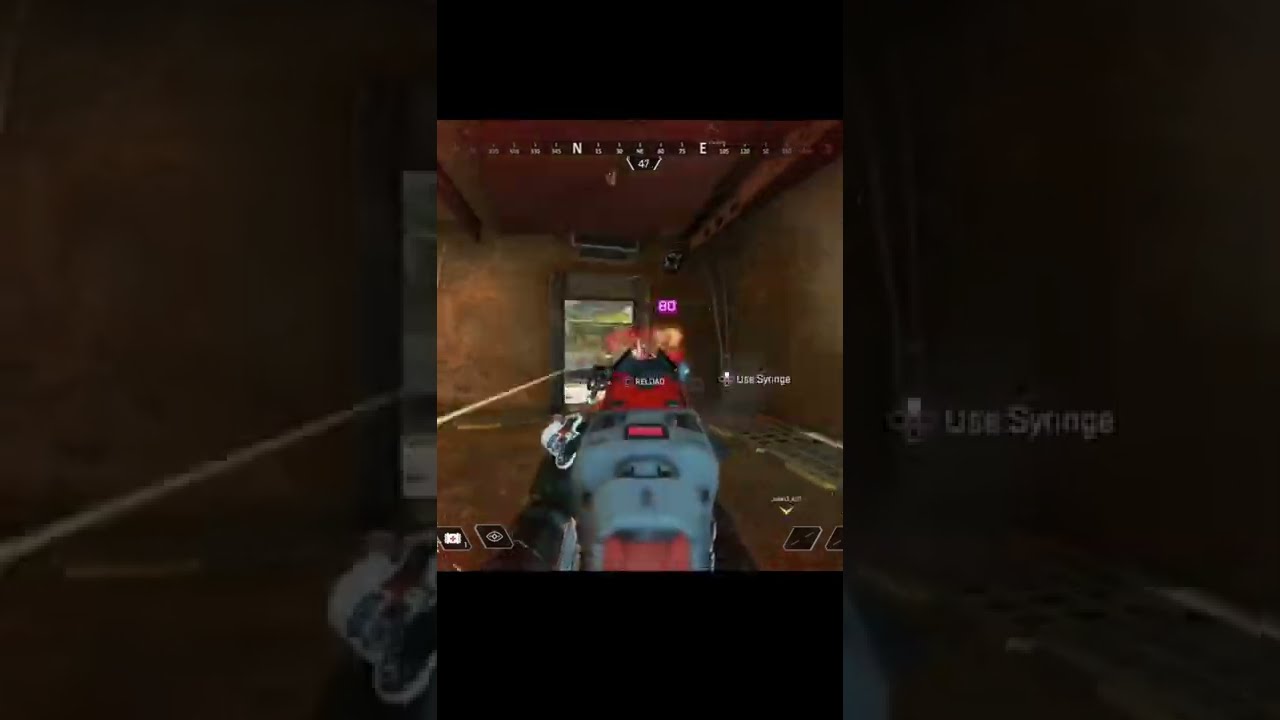The image appears to be a screenshot from an old first-person shooter video game, reminiscent of Doom. At the center is a small, square image set against a larger, faded background. The player's view features a gun, which is predominantly gray with a red tip, extending from the bottom center of the screen. The gun is pointed down a brown, dimly lit hallway, which could either be a spaceship corridor or a post-apocalyptic building. A light illuminates an open doorway at the end of the hallway, creating some distinction in an otherwise dark scene. 

To the right of this doorway, there is a magenta sign displaying the number "80." Just below the top section of the screen, a flatly-laid compass shows directional information, with 'N' and 'E' clearly visible. On the right side of the gun, a HUD keypad reads "Use Syringe," with the 'up' button highlighted in white. The screen also features some rhombus-shaped buttons on both the left and right sides, contributing to the navigational interface. While the overall image is underexposed and difficult to discern, these elements indicate a classic first-person shooter game setup.